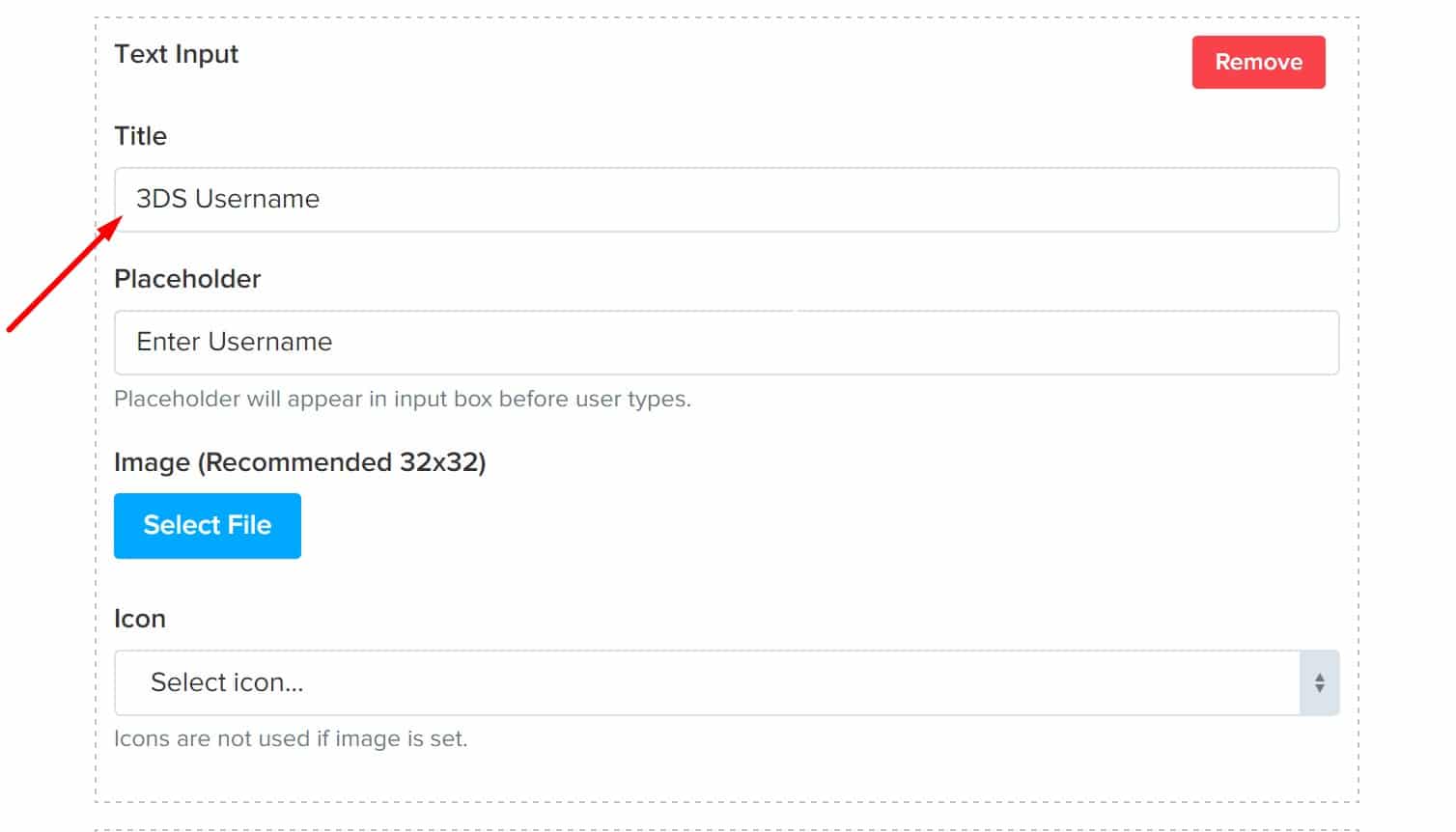The image displays a user interface form designed for input and customization. In the top left corner, there is a text input field labeled as "Text Input." The top right corner features a prominent red button labeled "Remove." Below these elements, a title field is present, pre-filled with the text "3DS Username."

Underneath the title, there is a placeholder text within the input box that says "Enter username," indicating where users should type their username. A smaller note below this box clarifies that this placeholder text will be displayed until the user begins typing.

Further down the form, there is a section designated for image upload. It suggests an image size of 32 by 32 pixels and includes a blue button that reads "Select File" for users to click and upload their image.

Next, there is an "Icon" section featuring a drop-down menu labeled "Select Icon." A note under this menu explains that selected icons will not be used if an image has already been set.

Overall, the image appears to illustrate a webpage form aimed at collecting and customizing a user's information, likely for a username setup or profile creation.